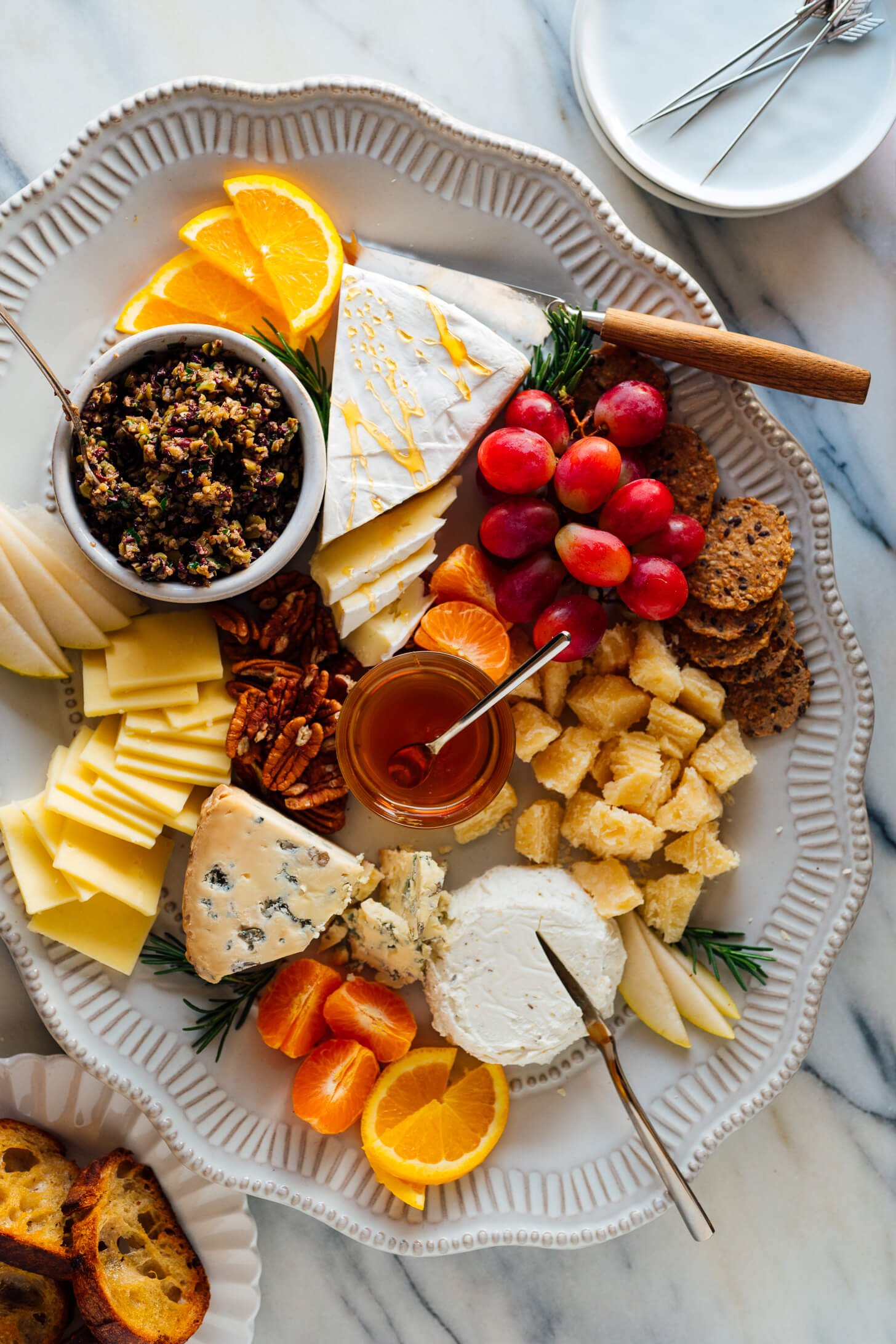This detailed photograph showcases a meticulously arranged charcuterie board presented on a large, white ceramic tray with gold trim. The tray features an array of visually appealing foods, neatly organized to entice any viewer. At the top, vibrant orange slices provide a colorful contrast. To the bottom right of these, a wedge of soft cheese – likely brie – is garnished with thin yellow streaks, possibly honey or another drizzle. Adjacent to this are small bowls filled with a variety of items: one contains a purplish-tan spread that resembles oatmeal, while another seems to hold a thick, raisiny dip.

To the left of the mysterious spread, ample slices of different cheeses are neatly assembled. Pecans are situated to the right of these cheese slices. Scattered around the board are various fruits, including smaller orange segments and what appear to be cherries or grapes. At the center of the arrangement, a small jar containing honey and a miniature spoon suggests a sweet addition to the savory items. Another cheese, possibly feta, is positioned nearby with a silver knife plunged into it for easy serving.

Further enhancing the variety, there are different types of crackers, some speckled with raisins or nuts, providing a complementary crunch. Also included is another plate featuring slices of bread, likely brioche, which is tan and inviting. Overall, this elegantly set up charcuterie board is a feast for the eyes and taste buds, emphasizing the harmonious blend of cheeses, fruits, nuts, and spreads.